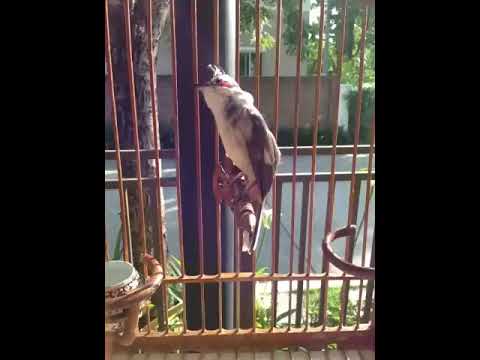The photograph features a bird with a white chest and belly, along with dark brown wings, perched inside an ornate birdcage. The cage, appearing to be of an orangey-bronze or gold color, is seen from a front angle with one of the bars slightly blurred against the lens, suggesting the picture is taken through the bars. The bird is captured in a left-side profile, stretching its neck up with the feathers on its head sticking up. Its wings and tail feathers are down. The cage is set against a black background, but through the bars and the window behind the bird, a residential neighborhood is visible. The view outside shows a clear, sunny day with green trees, well-manicured bushes, and a sidewalk or street, indicating a serene and pleasant environment.